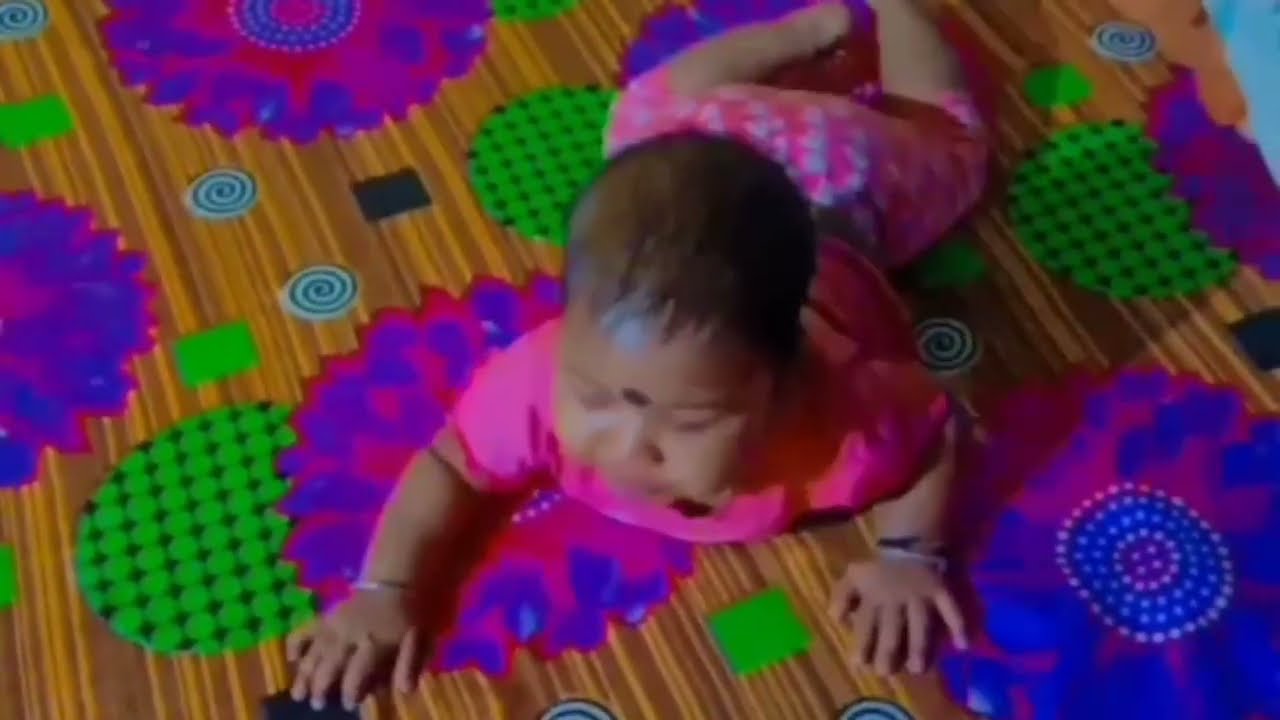This is a slightly blurred, horizontally-oriented photograph of a baby in the center of the image. The baby is crawling on a multi-colored floor mat composed of large, connectable pieces. The mat is decorated with various circular shapes, primarily in blue, purple, and green, with some having a small green diamond pattern. The baby, who appears to be about one year old, is positioned on her stomach, looking at something in front of her with her forearms on the mat and her legs stretched behind. She has short, black or dark brown hair and is wearing a pink short-sleeved shirt with patterned pink and white shorts. Additionally, she has two small bracelets on her wrists and a distinctive brown circle on her forehead, just above her nose. The background includes a wood grain tone interspersed with the colorful, geometric patterns of the mat. The style of the image suggests either a photograph taken with a cell phone or a freeze frame from a video, capturing the baby in a moment of exploration.